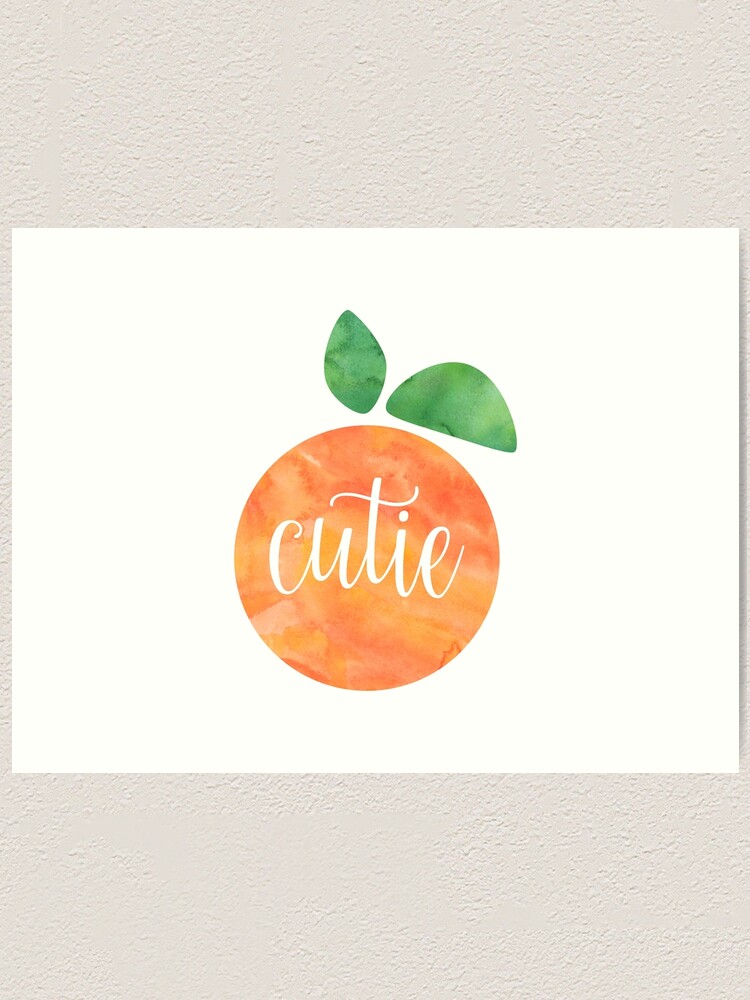This image features a close-up shot of an artistic postcard-sized white paper that showcases a detailed illustration of a circular orange. The orange, rendered with swirling hues of yellow, light orange, and blood orange, appears almost tie-dyed. Across the center of the orange, the word "cutie" is elegantly written in white lowercase cursive, with the 'T' slightly larger than the other letters. Above the orange, two green, oval-shaped leaves hover; one leaf points upwards while the other points downwards, adding a whimsical touch. The illustration is centered on a white, popcorn-textured wall with a surrounding cream-colored textured mat. The overall design is minimalistic yet charming, emphasizing the vibrant colors and neat handwriting.